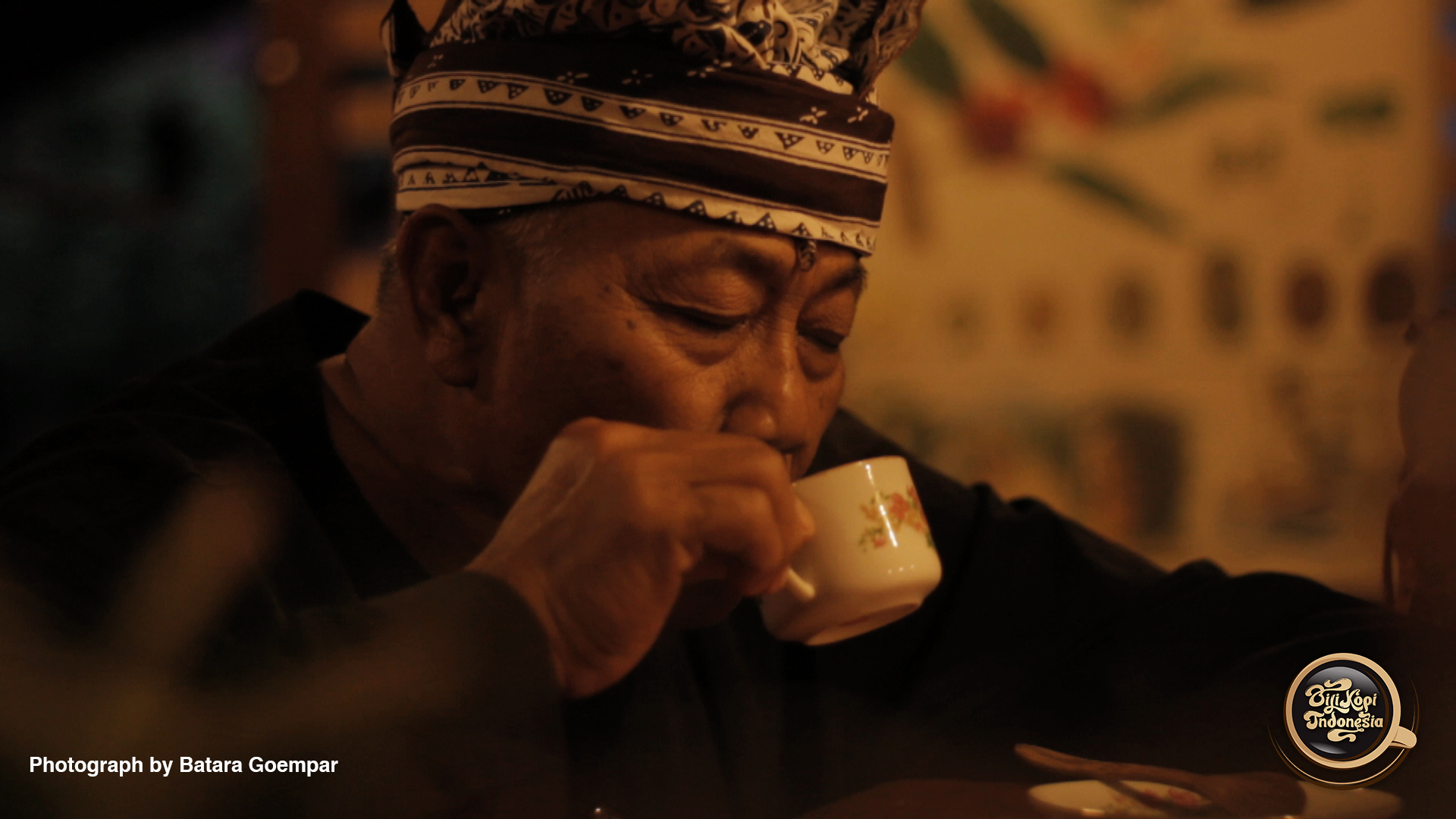In this candid photograph by Batara Duemper, an older man with dark, lined skin is pictured sipping from a small, white teacup adorned with flower patterns. The man, who has a flat, wide nose and is dressed in a black shirt, gazes intently into the cup, his right hand gently holding it. He wears a distinct black and white cloth hat featuring black triangular patterns on the white stripes. The softly lit image, likely captured indoors, frames him against a blurred backdrop embellished with leafy designs and red flowers, enhancing the intimate atmosphere. In the bottom left corner, the photo credits Batara Duemper, while a circular logo reading "BYRKOPF INDONESIA" appears in the bottom right, suggesting the photograph’s Indonesian cultural context.